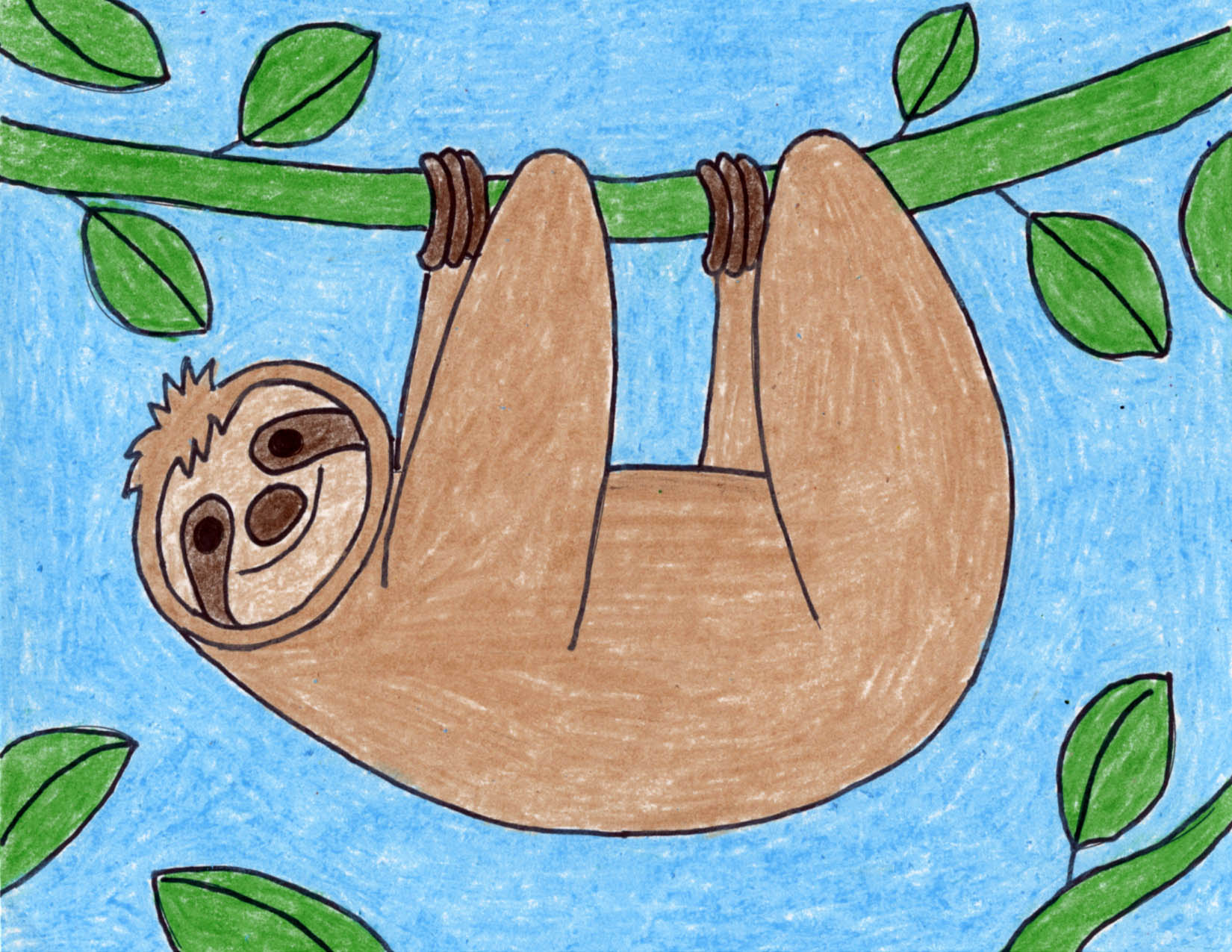This image is a simplistic and heartwarming illustration of a sloth, seemingly intended as a children's coloring page. The sloth is depicted hanging upside down from a green branch that extends horizontally from left to right, with a slight droop where the sloth's weight is attached. The branch is adorned with multiple leaves—three in the upper left-hand corner, two in the bottom left-hand corner, one in the bottom right-hand corner, and three, including one partially visible, in the upper right-hand corner. 

The sloth's body is colored in various shades of brown, with darker brown used for its claws and tufts of hair on its head. Its face is detailed with a tan and dark brown palette, and it sports a cheerful smile and beady black eyes. All four legs are wrapped securely around the branch, reinforcing its upside-down position with its back facing the ground.

The background is a sky-like blue, filled in with what appears to be colored pencil. Despite the intentional simplicity, the coloring maintains a neat appearance, staying largely within the lines but with deliberate gaps, giving it an authentic, handcrafted look. The illustration also includes a vine at the bottom, adding to the botanical theme.

Overall, the image conveys a sense of playfulness and charm, making it an engaging and delightful piece likely created for children.